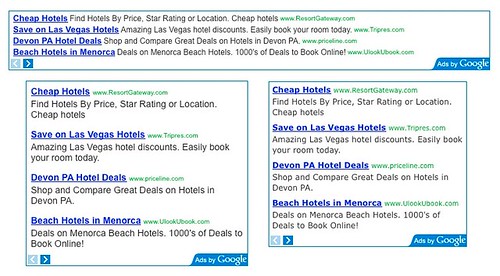In this image, you see a search results page displaying advertisements for various hotel deals. The page prominently features multiple lines of text repeated in different formats. At the top, there is an ad with the text: "Cheap hotels, find hotels by price, star rating, or location," followed by a link to www.resortgateway.com and a subheading promoting "Save on Las Vegas hotels: Amazing Las Vegas hotel discounts, easily book your room today."

Further down, another ad from www.tripest.com offers "Devon PA hotel deals: shop and compare great deals on hotels in Devon PA," followed by www.priceline.com advertising "Beach hotels in Manukau: deals on Manukau beach hotels, thousands of deals to book online."

At the bottom right, there's an "Ads by Google" label. The text "Cheap hotels, find hotels by price, star rating, or location" is repeated throughout the ads in different formats, laid out horizontally and vertically. The repetitive nature and varied presentation of this text highlight different aspects of hotel deals in multiple locations.